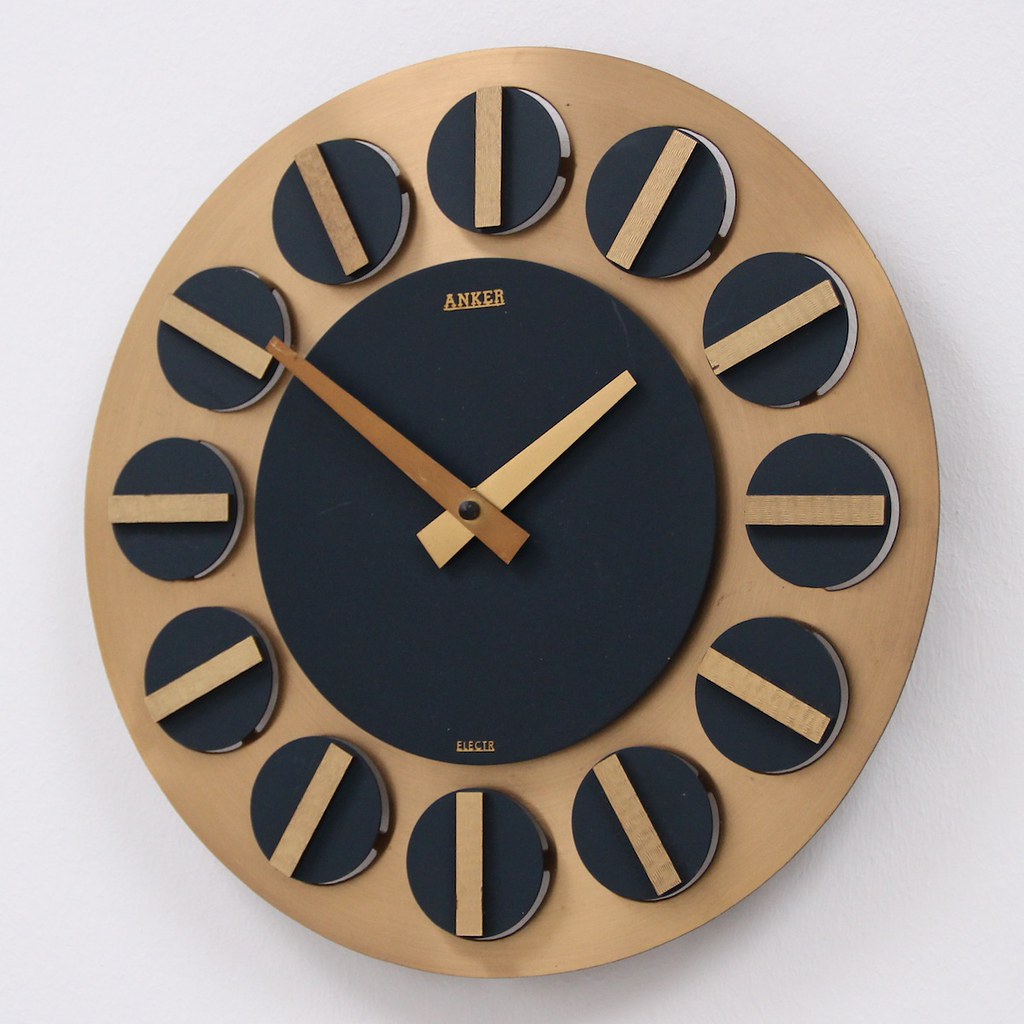This image depicts an elegant and distinctive clock. The clock features a circular frame with a golden brass finish. Instead of traditional numbers, it has black circular markers that are slightly elevated from the brass frame. Each black circle contains a brass line running through it and the word "Anchor" in brass lettering. The clock has two hands, an hour hand and a minute hand, both designed to complement the overall aesthetic. This beautifully crafted timepiece would make an impressive addition to any office.